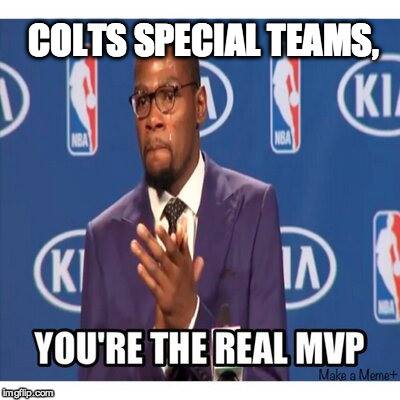The image is a meme featuring NBA player Kevin Durant standing in front of a backdrop with the NBA and Kia logos on a blue background. Durant is dressed in a purple suit with a white shirt, and he's wearing glasses. His eyes are tearful, and his hands are clasped together, creating a thankful or emotional expression. The meme text overlays the image with large white letters at the top saying, "COLTS SPECIAL TEAMS," and at the bottom saying, "YOU'RE THE REAL MVP." In the lower corners, smaller text reads "MAKE A MEME+" and "imgflip.com."